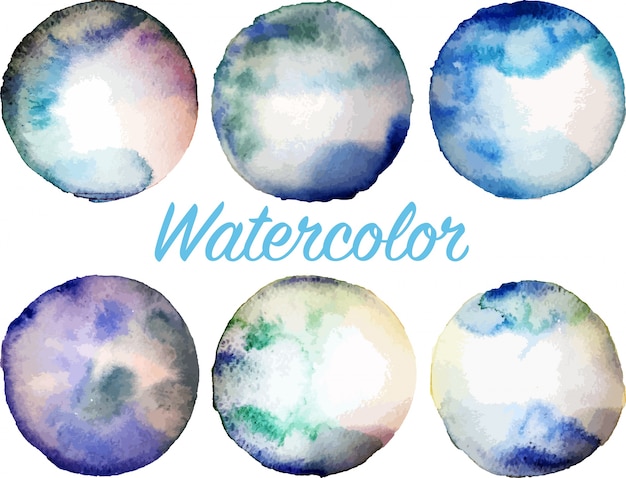The image presents six circular watercolor droplets arranged in a symmetrical layout against a white background, with three circles in the top row and three in the bottom row. At the center of the image, between the rows, the word “watercolor” is elegantly written in light blue script. 

Each droplet features a harmonious blend of colors that merge seamlessly together, creating a dreamy and fluid appearance typical of watercolors. Starting from the top left, the first droplet contains a mix of purple, blue, gray, black, and white. Moving to the middle of the top row, the second droplet showcases shades of blue, green, and white. The final droplet on the top right displays a combination of dark blue, lighter blue, and white.

On the bottom row, the first droplet on the left integrates light and dark purple with green, gray, and white. The middle droplet primarily features white with accents of green and blue. The last droplet on the bottom right displays a dominant white center surrounded by blue-green hues, light and dark blue colors.

Collectively, these droplets transition through a spectrum of colors from violet to blue and green, creating a cohesive and visually appealing ensemble.